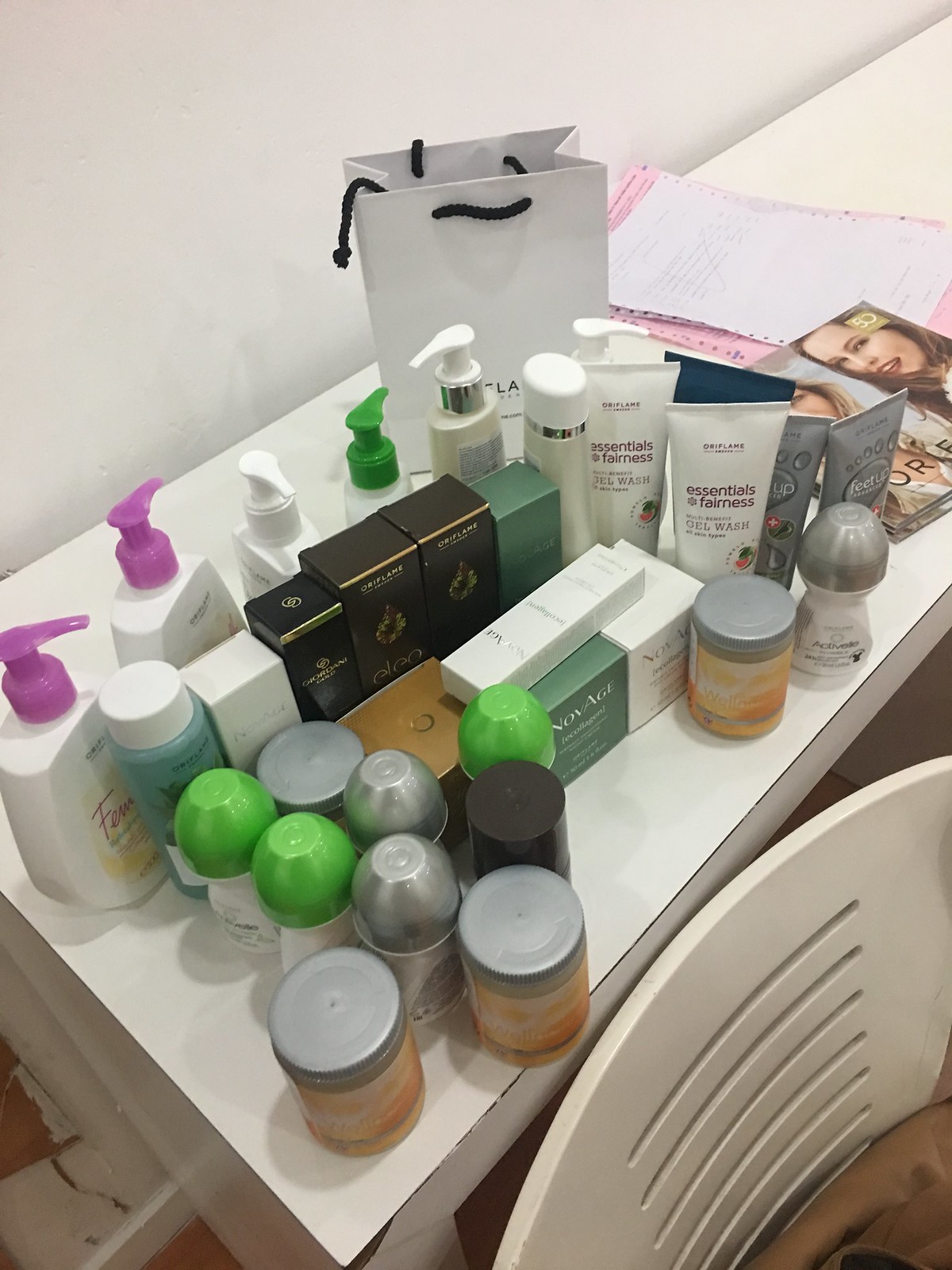The image showcases a minimalistic setup against a white wall. Pressed against this wall is a white table, with a distinctive white chair in front of it. The chair features horizontal cut-out lines on the backrest. On the floor to the left of the table is a box.

On the tabletop, towards the far right, lies a pink piece of paper with a white piece of paper placed atop it. Adjacent to these papers, there is a white bag with a black string handle. Below the table, several plastic bottles with pumps are visible, with pumps in various colors: purple, white, and green. In front of these bottles, there are cardboard cartons in black, white, and green.

To the right of these cartons, several tubes stand upright with their caps facing downward. Further to the left, additional plastic containers can be seen, with tops in green, gray, and black hues.